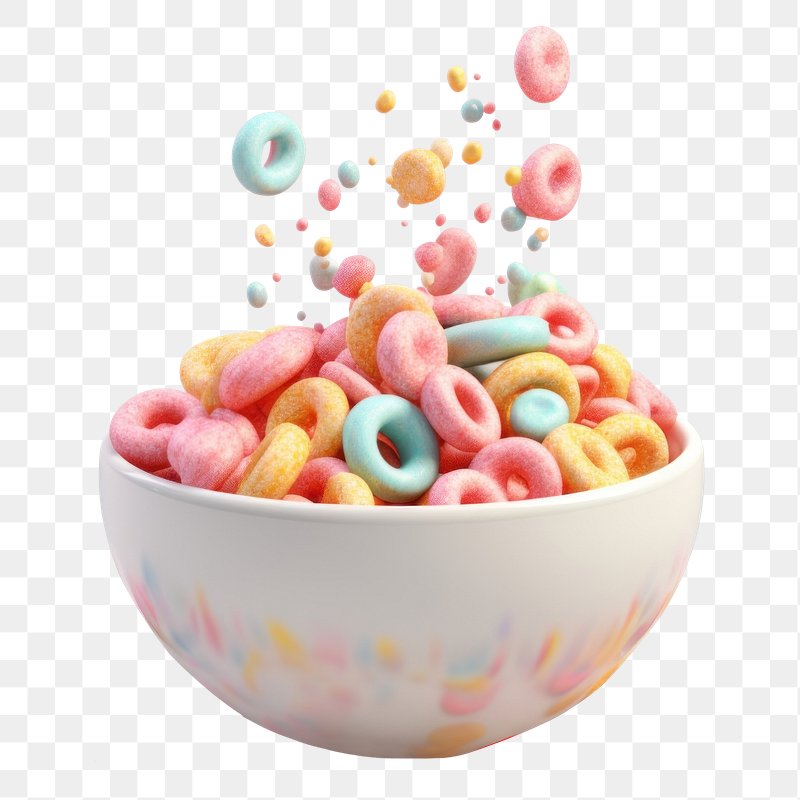In the image, a bowl of colorful, donut-shaped cereal, reminiscent of Cheerios but in colors like pink, orange, and blue, is set against a light gray and white checkerboard background. The checkerboard pattern is denser than a typical one, featuring approximately 30 squares across and 30 squares down, creating a vibrant backdrop. The white bowl itself is adorned with small splotches of the same colors found in the cereal, particularly towards its bottom. The cereal overflows the bowl, with a cascade of loops seemingly suspended in mid-air above and around it, giving the impression that it is raining these colorful loops. Amidst the rain, some of the loops are fully intact while a few exhibit an indentation in the middle without a complete hole. The background pattern appears darker at the top, gradually lightening towards the bottom, further enhancing the whimsical, floating effect of the cereal pieces.